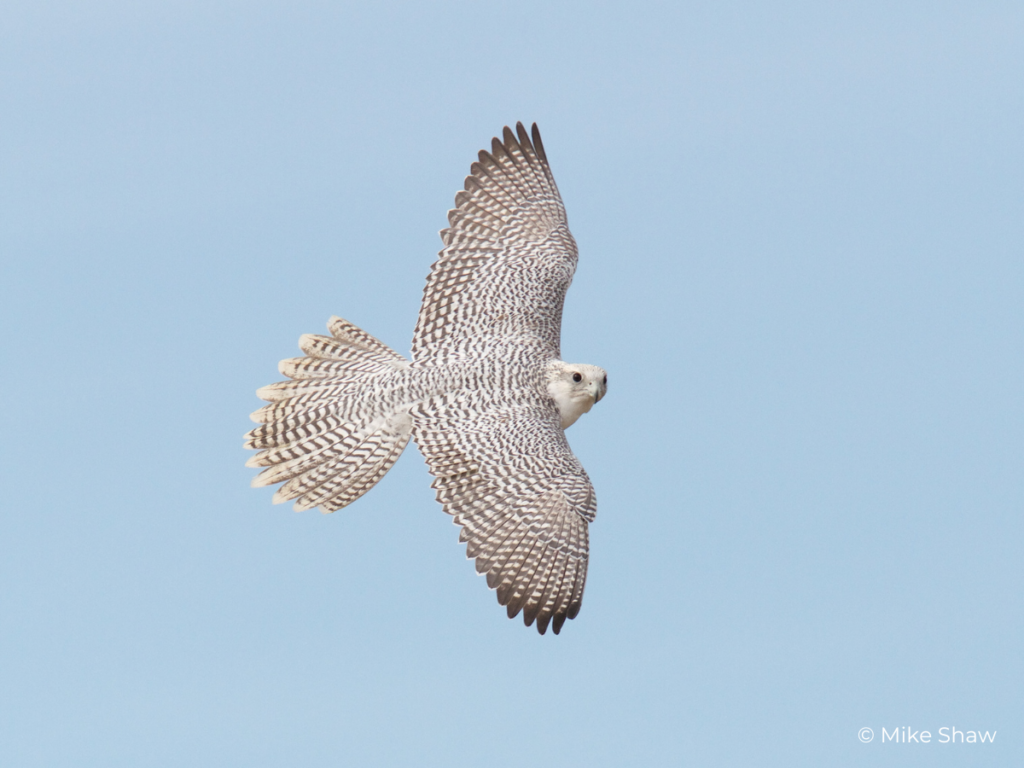This captivating photograph, taken by Mike Shaw and copyrighted under his name, features a majestic raptor, likely a hawk, soaring through the sky. The bird, which displays intricate white and brown plumage with a strikingly white head, appears mid-flight in the clear, cloudless blue sky. Its left wing is tilted upwards towards the camera, while its right wing angles downwards, capturing a dynamic moment possibly assisted by a drone's perspective. The hawk's keen eyes are locked onto the lens, exuding a sense of confusion and curiosity as if it is unsure of its next move. The sharp beak and intense gaze further enhance the predatory nature of this beautiful bird. The overall scene is framed with immaculate detail, highlighting the contrasting baby blue sky and the bird's darkened wingtips, a testament to Shaw's delicate and skilled photography.